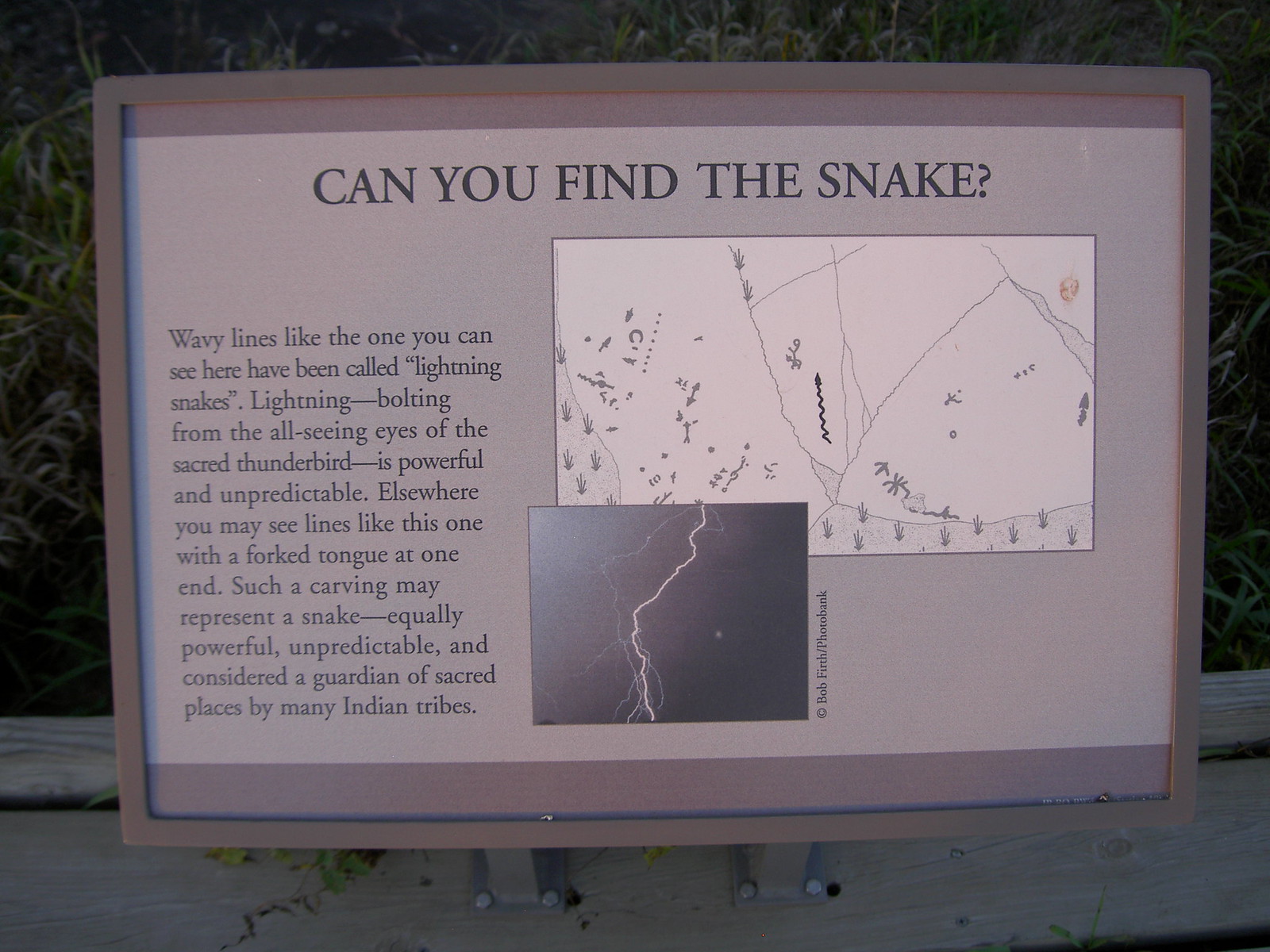The image shows a plaque bordered with a grey frame, likely situated on a wall in a park or along a trail. The top of the plaque features a title in black text that reads, "Can you find the snakes?" To the left, there is descriptive text about wavy lines, explaining that these have been called "lightning snakes," representing lightning bolting from the all-seeing eyes of the powerful and unpredictable sacred Thunderbird. It further mentions that elsewhere, similar lines might appear with a forked tongue at one end, symbolizing a snake that is equally powerful and unpredictable, often considered a guardian of sacred places by many Indian tribes. The right side of the plaque includes images—an aerial map resembling a trail, and a photograph of a lightning bolt credited to Bob Firth from Photobank. The entire plaque is mounted onto a wooden beam.